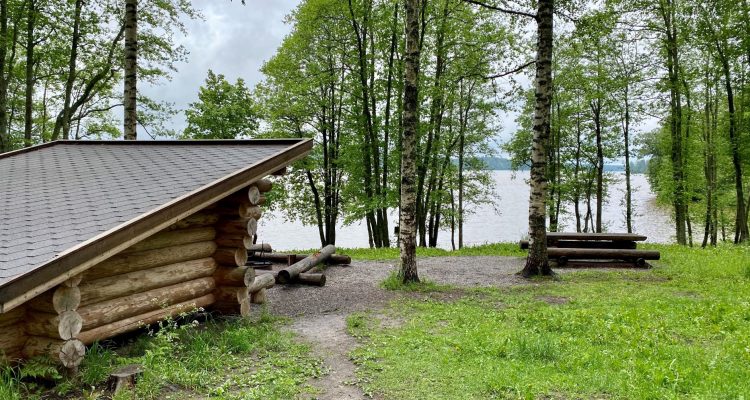This photograph captures an outdoor setting dominated by an overcast sky filled with clouds. The ground area at the bottom of the image features patches of green grass interspersed with dirt. On the left side of the scene stands a quaint, small wooden log cabin with a flat, grayish roof. Just outside the cabin, there are several wooden logs placed on the ground, which is mostly gray. The cabin appears lower to the ground, adding a rustic charm to the setting. To the right, a wooden bench is placed amongst the many trees, which have thin trunks and contribute to the natural atmosphere. In the background, a body of water stretches across the horizon, bordered by more trees that partially obscure the sky.